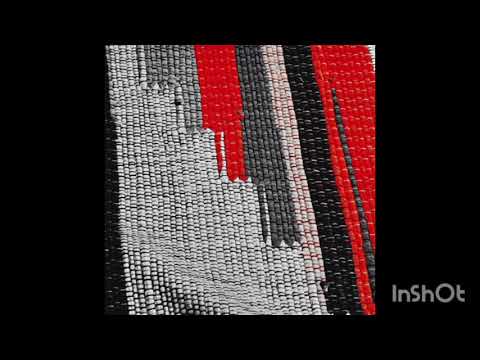The image depicts a highly detailed, macro photograph of a fabric, possibly a floor or table mat, set against a stark black background. The fabric occupies the center of the image, featuring intricate stitching that showcases its texture up close. The color palette includes black, light gray, dark gray, red, and white. A striking large red stripe runs vertically on the right side of the fabric, accompanied by thinner gray and black lines. Adjacent to these is a sequence of stripes: a white line, a dark gray line with a gap at the bottom, a slightly shorter red line, and a light gray line. The fabric appears to have layered yarn that creates the impression of depth and complexity. In the lower right-hand corner, the text "in shot" appears in gray. The photograph is cropped closely, making it difficult to discern the fabric's precise use, although it may be placed on a kitchen table.